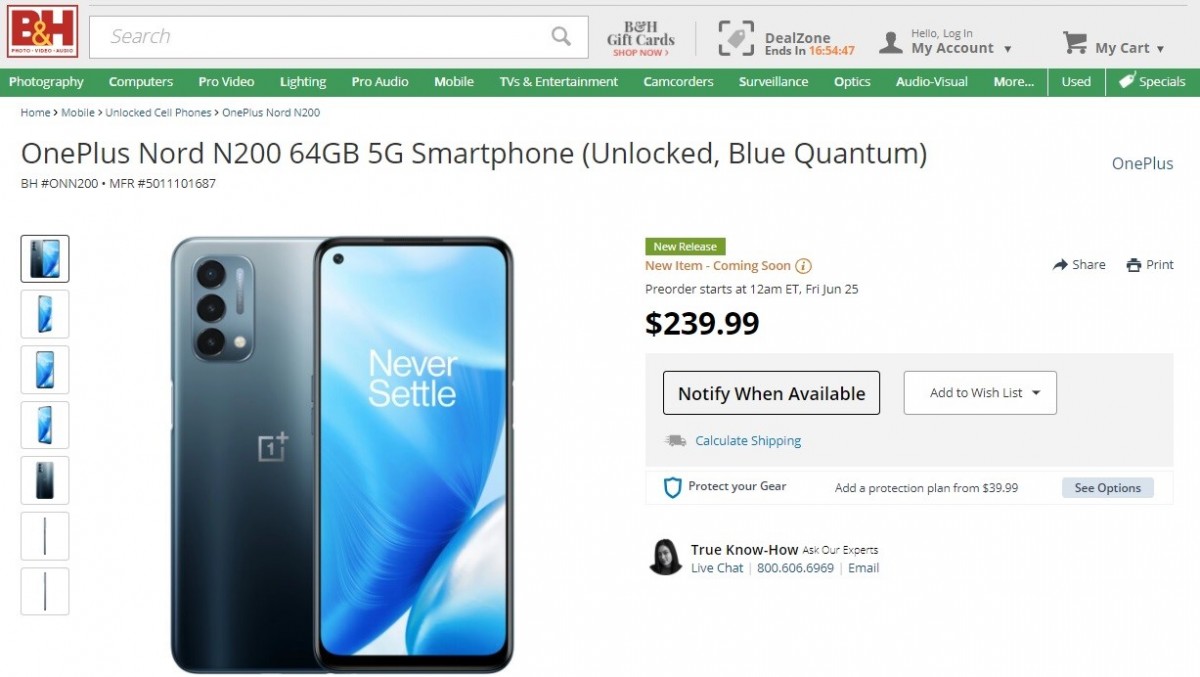Screenshot of a Website Interface:

The screenshot captures a portion of a web page that prominently features the branding and various navigation elements of the site. Starting from the top left, the image includes a logo consisting of a red rectangle with capital letters "B" and "H" in white, separated by a golden "and" symbol in the center. Directly below the logo, the partially visible text reads "photo-video-AAAUS," though the end is cut off and slightly blurred.

To the right of the logo is a dark grey bezel. Featured on this bezel is an advertisement for B&H gift cards, with the text "B&H Gift Cards" and a "Shop Now" button in red, accompanied by a right-pointing arrow also in red. Adjacent to this, there is a "Deal Zone" label with a time countdown (in orange) showing "ends in 16:54:47."

On the right side of the screen, there is a silhouette of a person labeled with "Hello, Login" next to a "My Account" dropdown menu, followed by a cart icon labeled "My Cart."

The main part of the screen includes a navigation bar with blue links stating "Home" and "Mobile Unlocked Cell Phones." Beneath the navigation bar, the product section highlights the "OnePlus Nord N200 G4 5G Smartphone," labeled in bold black text with the description "(Unlocked, Blue Quantum)" in parentheses. Below this product title, a green rectangle with white text marks the item as a "New Release," and additional brown text states "New Item - Coming Soon" accompanied by an information icon.

Further details about the product include a reorder date and time ("Reorder starts at 12am Eastern Time Friday June 25th") and a price of "$239.99." Two call-to-action buttons are located below the price: a dark grey "Notify Me When Available" button with black text, and a white "Add to Wish List" button, the latter featuring a dropdown menu without visible options.

On the left side of the screen, another blue link displays "Calculating Shopping." At the bottom left, there is a black and white profile picture of a woman with shoulder-length hair next to the partially obstructed text "true no-how" and thinner black text "escrow exports." At the bottom right, contact options including "Live Chat," a phone number (800-606-6969), and an "Email" link are listed.